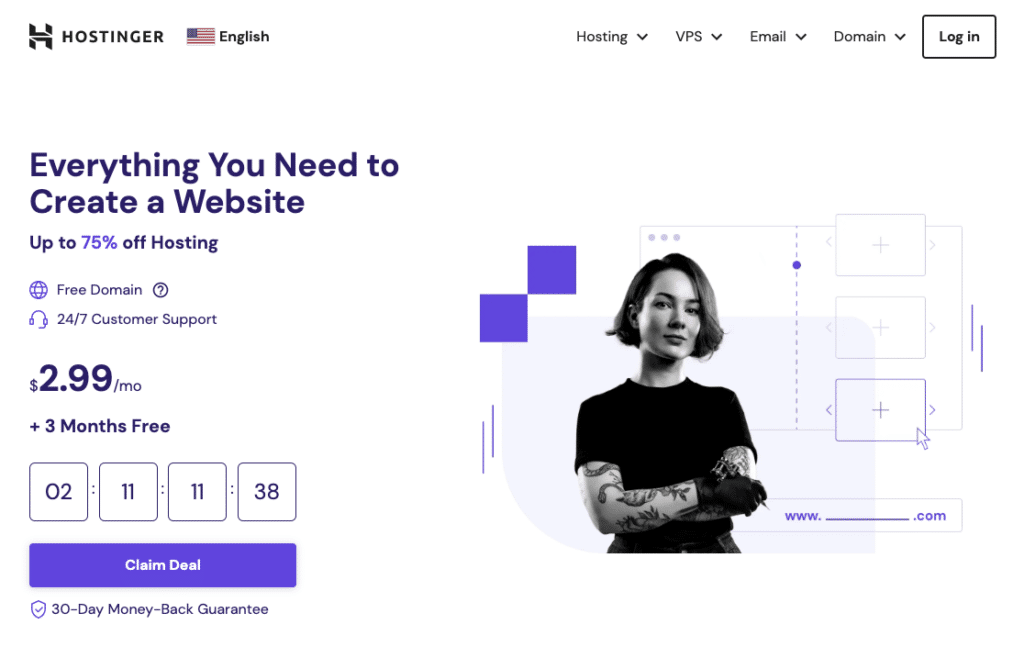A detailed screenshot of a web hosting service's promotional webpage. The top section features a vibrant banner with an image of a popular singer associated with the brand. Adjacent to it, there is an American flag icon indicating English language support. The navigation menu offers options such as "Hosting," "VPS," "Email," "Domain," and a prominently highlighted "Login" button enclosed within a rectangle.

The main promotional content informs users that they can create a website with up to 75% off on hosting services, with the "75%" discount figure displayed in bold blue text. There is a mention of a "Free Domain" offer, marked with a question mark inside a circle for more details. The webpage also highlights 24/7 customer support.

A prominent price display lists the service at $2.99 per month, with an additional offer of three free months included. A countdown timer below shows "2 days, 11 hours, 11 minutes, and 38 seconds" left to claim the deal, suggesting urgency. 

At the bottom, the webpage assures users with a "30-Day Money-Back Guarantee." To the right of this section, there is an image of a woman, possibly symbolizing customer satisfaction or support.

The footer contains the URL "www.example.com" in blue text, standing out against the rest of the content.